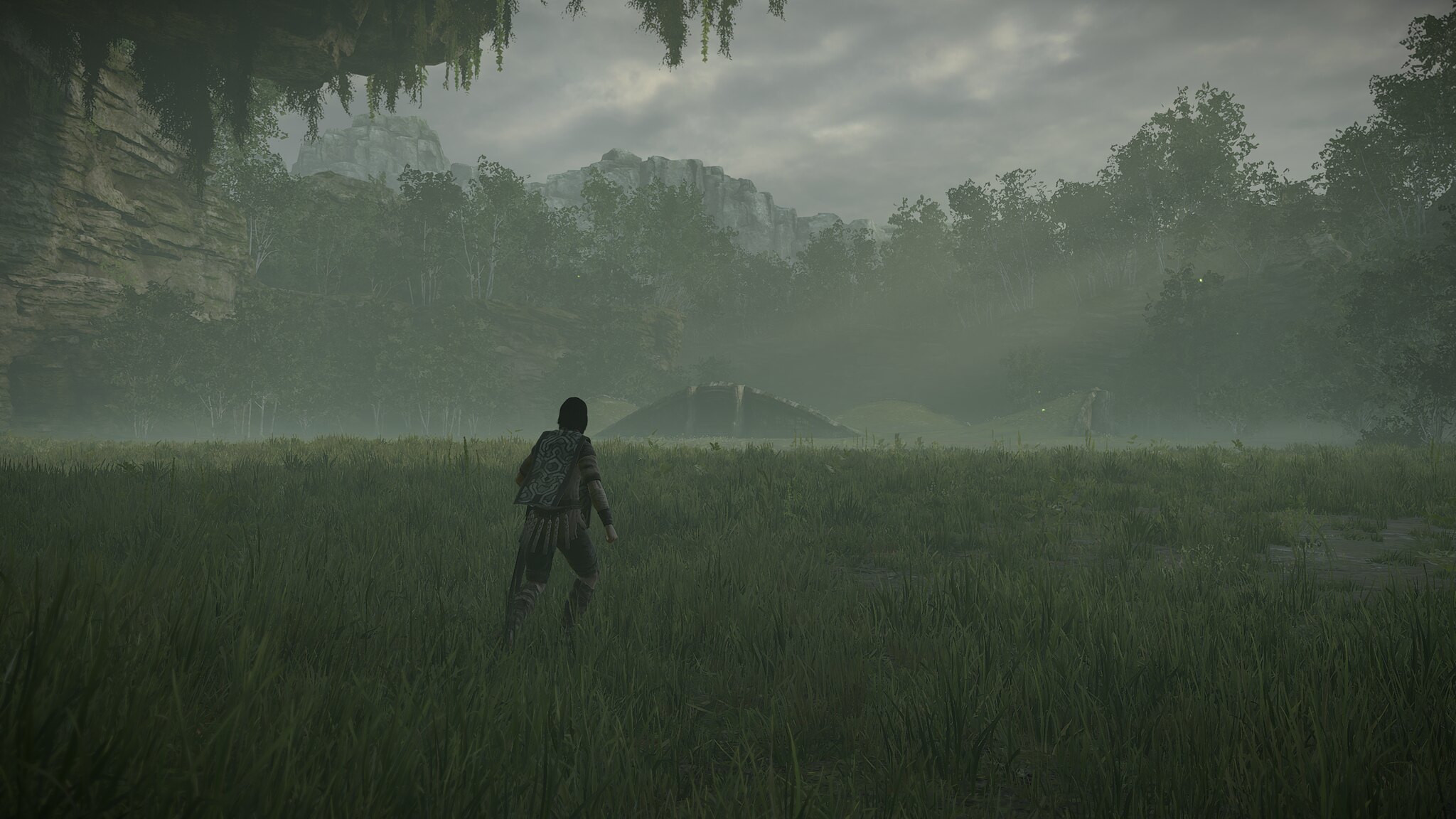In this evocative image, the composition highlights a solitary figure standing in the foreground, gazing intently toward a distant, mountainous, and forested backdrop. The scene is suffused with a palette of greenish and bluish hues, reinforcing the misty, overcast atmosphere created by the cloudy sky. The weather is distinctly foggy, adding an ethereal quality to the landscape.

The individual in the foreground, potentially a male, is clad in dark clothing and carries a backpack, though their exact identity and race remain ambiguous. They stand on an overgrown field, with ankle-high green grass swaying gently around them. The attention to detail captures the rugged, untamed nature of the terrain.

In the distance, towering trees and mountain peaks dominate the horizon, shrouded in a blanket of mist that blurs their outlines. The photograph also subtly includes the delicate overhang of what appears to be willow branches or moss-covered trees at the fringes, contributing to the lush, verdant theme.

This captivating image, suffused with a blend of green, blue, and white tones, beautifully captures the mood of a serene yet mysterious wilderness. It invites viewers to share in the quiet contemplation of the solitary figure, as they stand in awe of the natural beauty surrounding them.